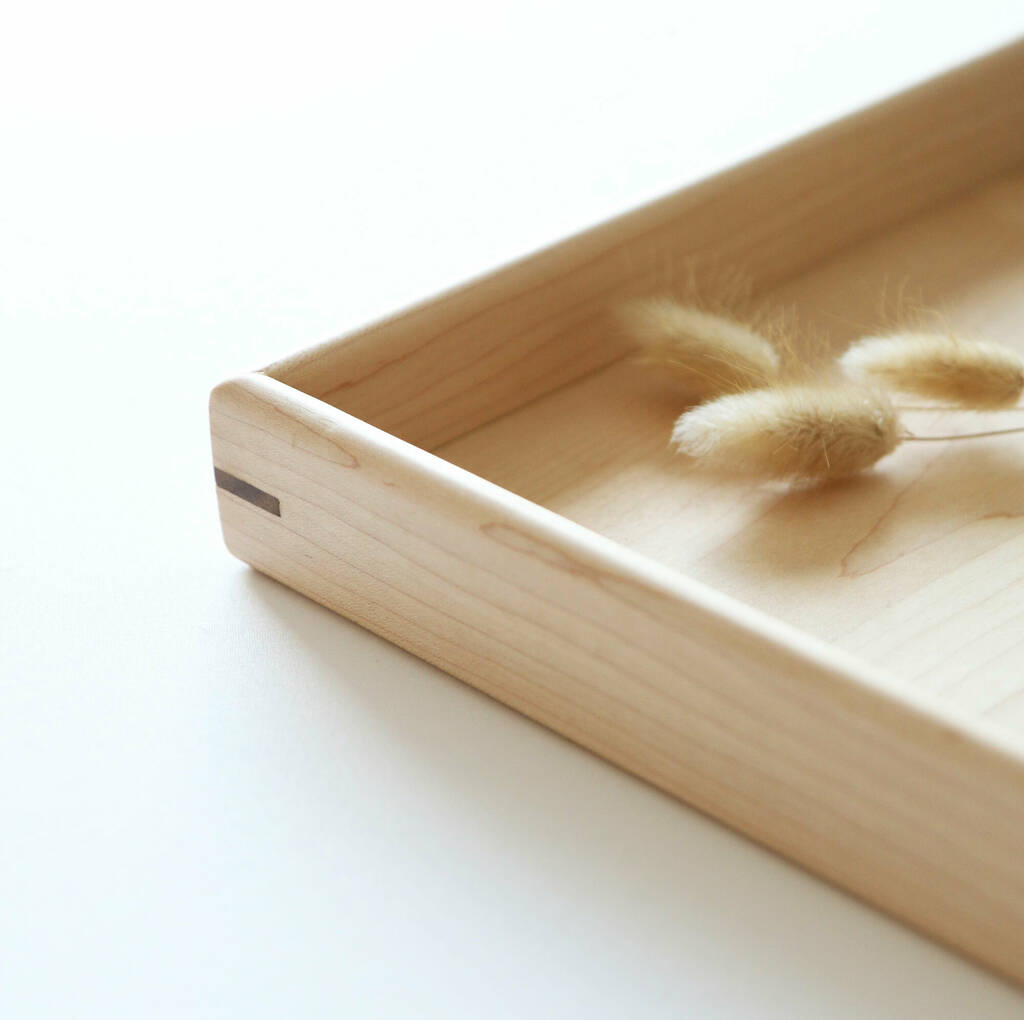The image presents an exquisitely crafted wooden tray corner, predominantly light tan or white in color. The tray, which appears to be approximately an inch to an inch and a half deep, features smooth, sanded edges and is reinforced at the corners with darker-colored wooden pegs, showcasing its meticulous construction. Inside the tray, positioned in the lower corner, are three fluffy, light tan to white pussy willows. These elegant, fuzzy plants resemble the delicate texture of dandelions and add a natural, decorative element to the simple yet stylish tray. The background of the image is a clean, light gray or white, providing a neutral backdrop that highlights the tray and its contents.